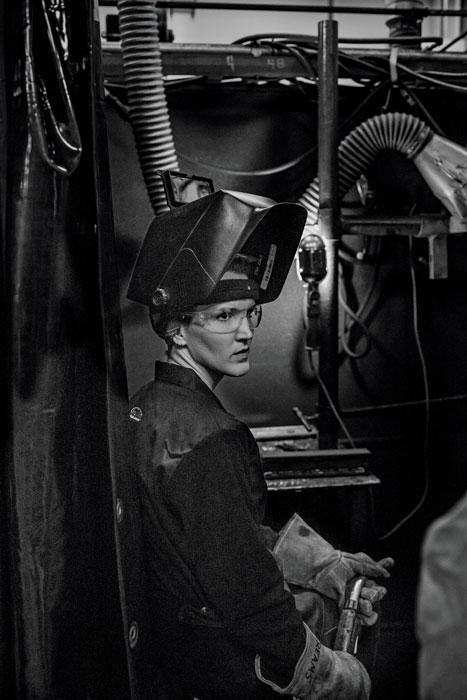The black-and-white photograph depicts a young welder, identifiable by a helmet pushed up to reveal his face adorned with safety glasses. He is a white male wearing a black shirt, jumper suit, and thick leather gloves. His head is turned to the right, directing his gaze outward. The welder holds a metallic object, potentially a tool or screw, in his right hand. Positioned in a dimly lit, industrial setting, the background showcases an array of tubing, cables, and pipes against a dark gray backdrop. A portable work light, affixed to a structural pole and turned on, serves as the brightest element in the image. The composition also includes a glimpse of another person's shoulder and suggests a two-floor environment with various industrial fixtures.